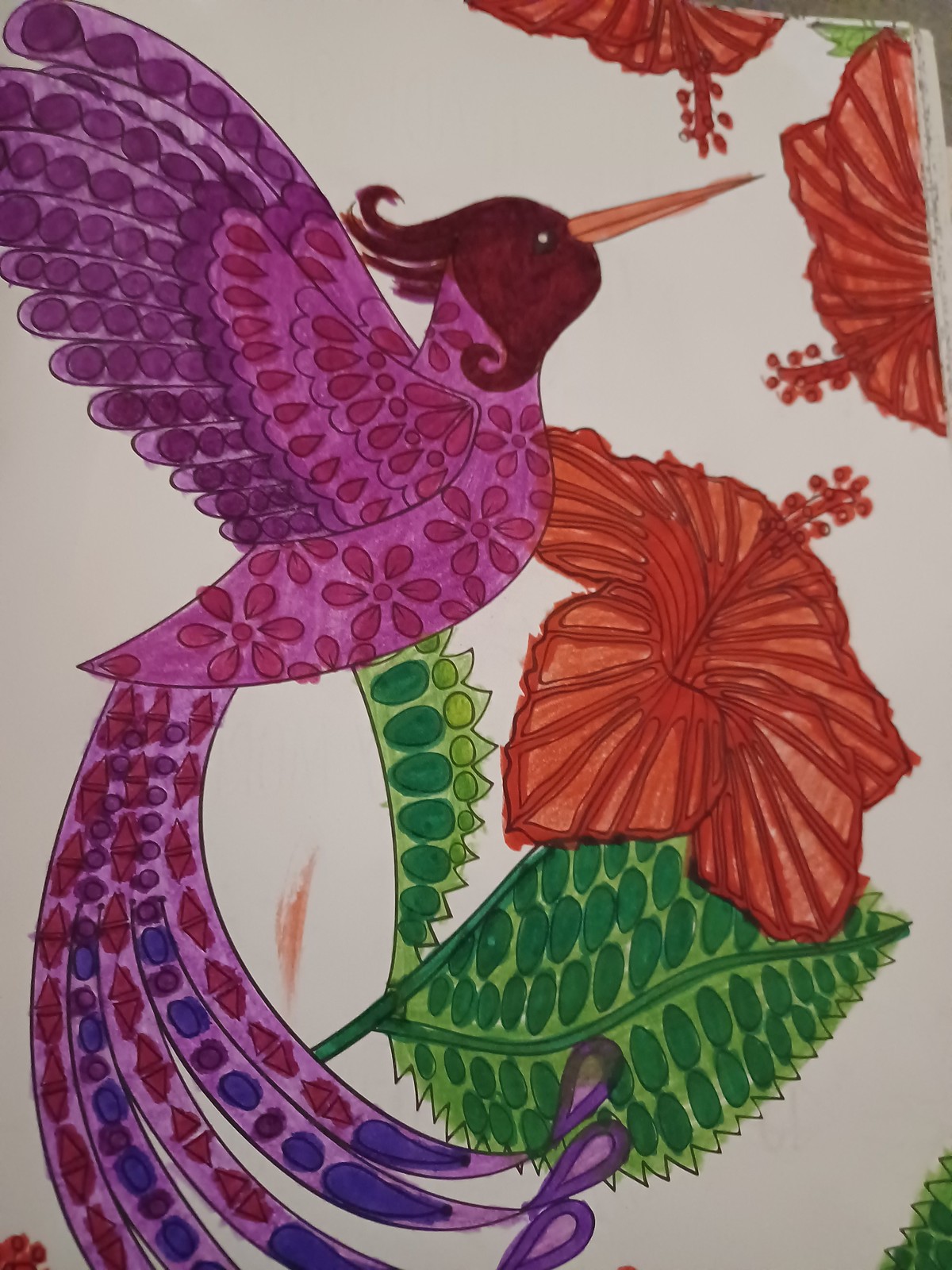The image depicts a vibrant and intricately colored drawing of a hummingbird engaged in feeding from three large, red flowers. The hummingbird, predominantly adorned in shades of purple and maroon, features a long, striking orange beak, and its face is of a deep, burnt red hue. The bird’s body is elaborately decorated with floral patterns, while its wings showcase a variety of circular and oval designs in purple. The tail, extending gracefully down the picture, is adorned with diamond-shaped patterns and includes hues of bluish purple.

The bird, which occupies the majority of the canvas-like background, is set among an array of foliage. Below the bird’s breast, a prominent green leaf with numerous dark green circular designs adds to the scene’s rich detail. To the upper right of the hummingbird, the three sizable flowers, colored in deep reds and oranges, are partially visible, with two extending beyond the frame and the third positioned just below the bird. The entire composition seems to be rendered with markers, characterized by vivid colors and detailed patterns, creating a visually stimulating piece. A small scribble mark is also noticeable between the bird’s tail and the green leaf.